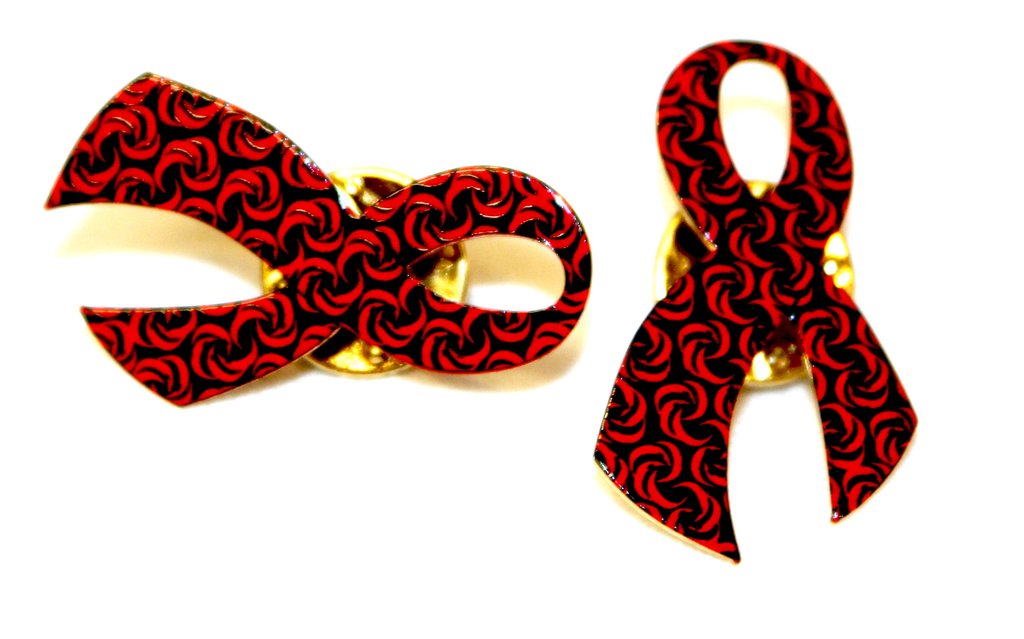The image is a close-up photograph with a white background, showcasing two decorative pins prominently positioned in the center. Each pin features a ribbon-like design with a black and red swirl pattern, forming a loop and creating an open figure-eight shape. One pin is oriented vertically, while the other is placed horizontally, seemingly crisscrossing each other. The base of each pin is a shiny, circular gold back piece that secures the ribbons in place. The overall appearance is clear and bright, with no additional objects, text, or numbers present in the photograph, accentuating the intricate details of the pins. The clarity and natural lighting highlight the elegant, intertwined ribbon design and the lustrous gold bases.